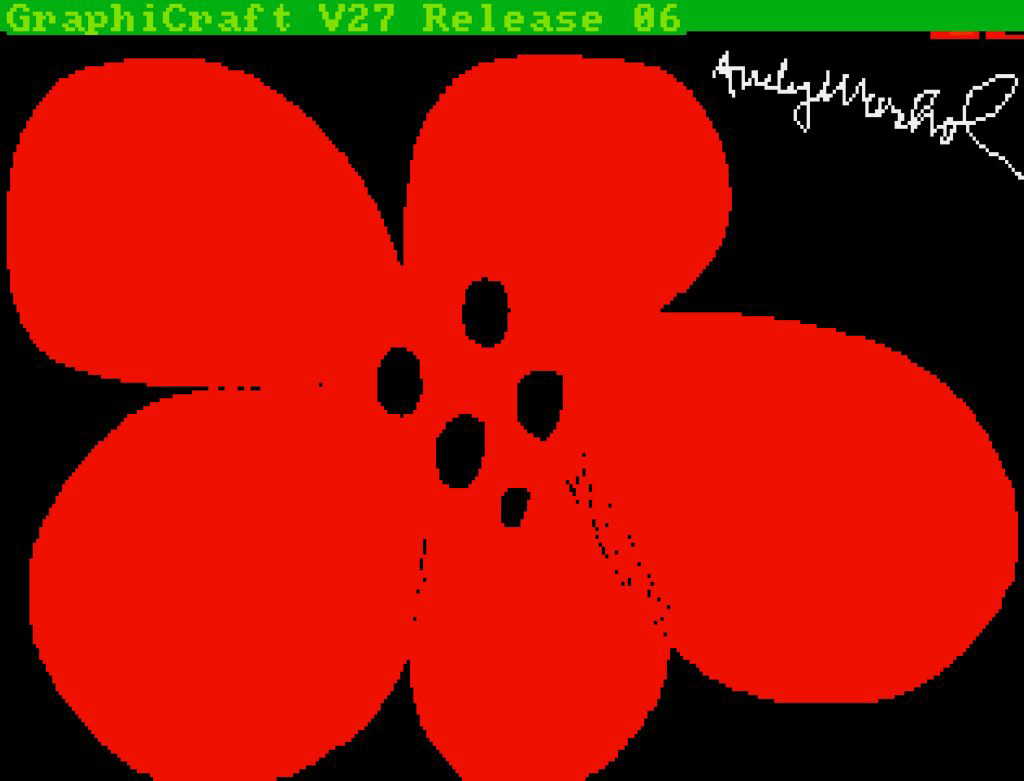The image depicts a simplistic, computer-generated drawing, reminiscent of a childlike style. Central to the composition is a large red flower with five petals, each petal radiating from a center adorned with five black dots. Additional smaller black dots are scattered on the lower left and right sides of the flower's center. The background is a solid black, creating a stark contrast with the vibrant red of the flower. In the upper right corner of the image, there is an artist's autograph in white, though it is difficult to decipher. Above the black background, a thick green banner stretches horizontally across the top, inscribed in a lighter lime green font with the text, "Graphicraft V27 Release 06." The banner slightly overlaps with the artwork, touching the red petals of the flower. The image appears to be a basic digital graphic exercise, likely created using a mouse, indicating an introductory level of proficiency in computer art.